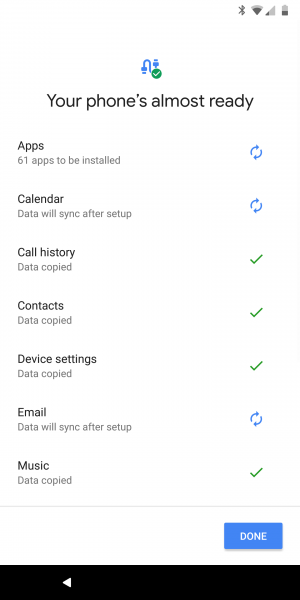This screenshot, captured from a mobile device, depicts a stage in the phone setup process where data is being transferred, likely from an old phone to a new one via cloud synchronization. At the top of the image, a message reads, "Your phone's almost ready," indicating the nearing completion of the setup. The top of the screen shows standard smartphone icons such as Bluetooth connectivity, Wi-Fi signal, network status, and battery life. Below the message, a detailed list displays various categories of data being transferred: apps, calendar, call history, contacts, device settings, email, and music. Each item in the list is accompanied by a status indicator - a green tick for completed transfers and two arrows circling each other for items currently being copied or pending synchronization.